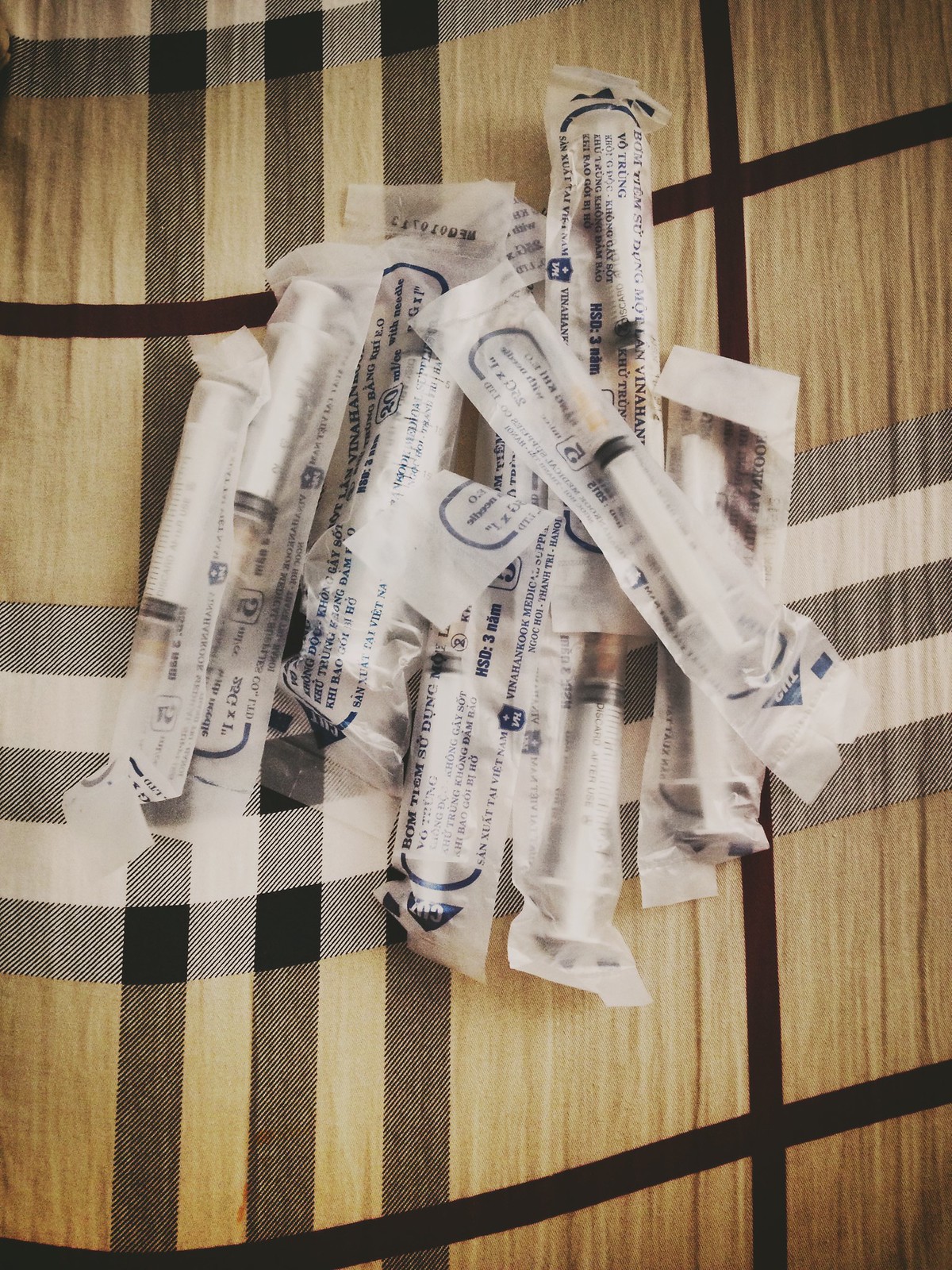This image showcases a collection of sealed syringes piled haphazardly on a checkered fabric backdrop. The syringes, which appear to be small needles, are encased in clear plastic packaging, revealing a white plunger and a black ring around the base of each syringe. The packaging features labeling in a foreign language written in black text. The syringes are mostly arranged parallel to each other, some overlapping, with one positioned diagonally atop the others. This assembly lies on a material with a distinct pattern: a mix of black and white plaid on a tan background interspersed with several dark horizontal and vertical stripes, suggesting a soft fabric such as a blanket or throw. The image captures the intricate contrast between the transparent sterile packaging of the syringes and the textured, patterned surface they rest upon.